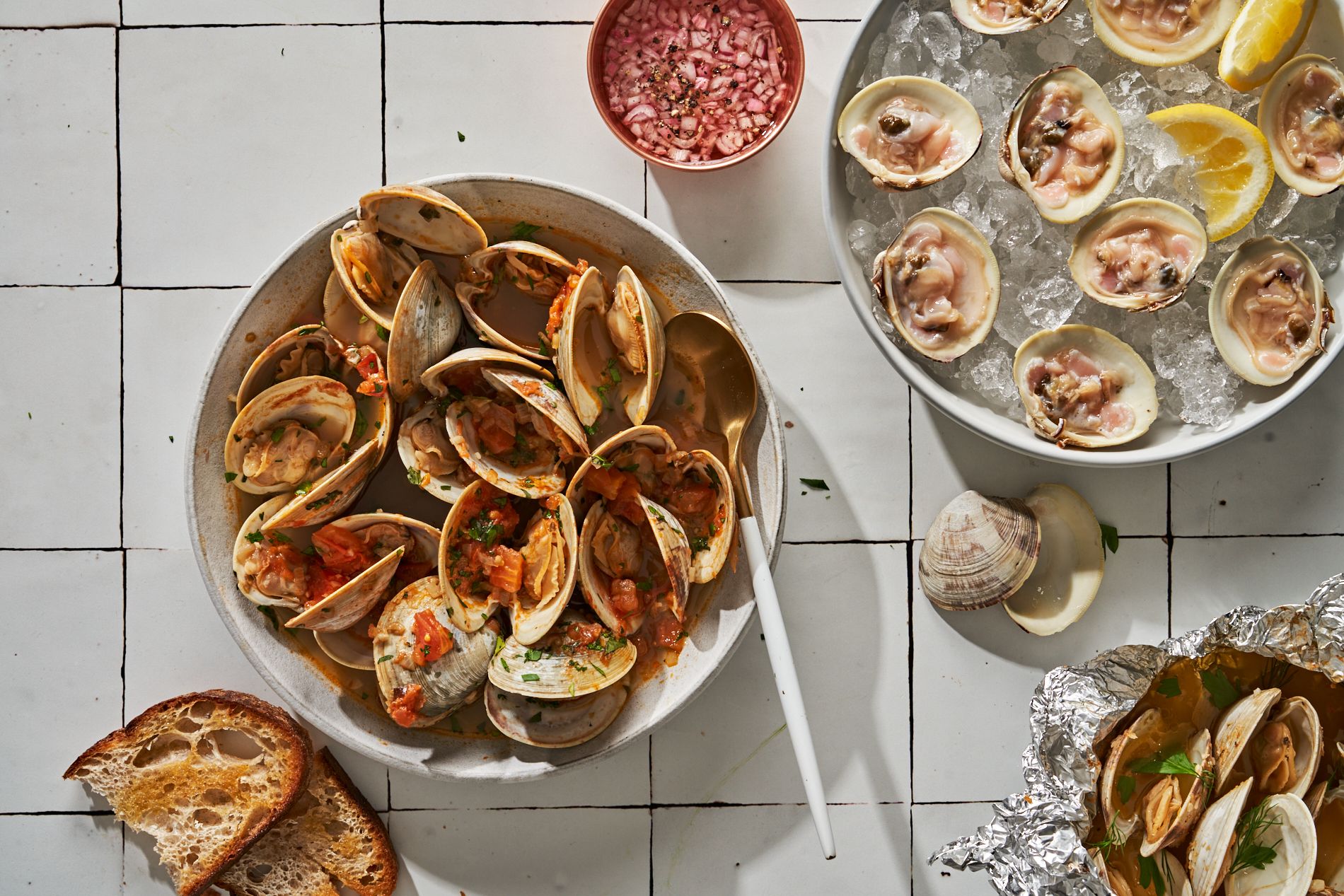In this detailed photograph, several food items are artfully arranged on a white tiled countertop accented with black lines. Prominently featured are various preparations of oysters. On the top right, a bowl filled with fresh oysters sits on a bed of ice, accompanied by lemon slices for garnish. The middle right showcases an assortment of sautéed oysters draped in a rich sauce, served in a white bowl with a white-handled spoon standing ready for serving. Nearby, an empty oyster shell rests solo, emphasizing the focus on these delicacies.

Towards the bottom right, a collection of oysters, seemingly baked or sautéed with sauce, are neatly assembled in an opened foil wrap. On the bottom left, two slices of perfectly toasted bread, possibly garlic bread, add a complementary texture to the seafood. A small red cup containing a sauce or condiment sits at the top, ready to enhance the flavors. The setup, devoid of any text, draws attention solely to the deliciously inviting food presentation.